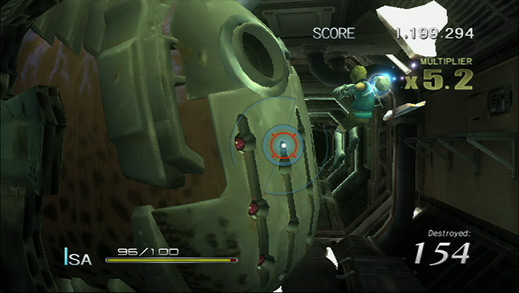A rectangular screenshot from a video game, featuring vibrant, cartoonish graphics. Prominent in the scene is a green object with brown spots along its side. At the top of the image, the score "1,199,294" is displayed in white text, accompanied by a multiplier reading "X5.2." To the right of the score, a little cartoon man appears to be floating in zero gravity. At the bottom of the screen, the text "Destroyed: 154" is clearly visible. On the left side, "ISA" is written next to a bar with a green indicator reading "95 out of 100." The overall visuals suggest a setting inside a space capsule.